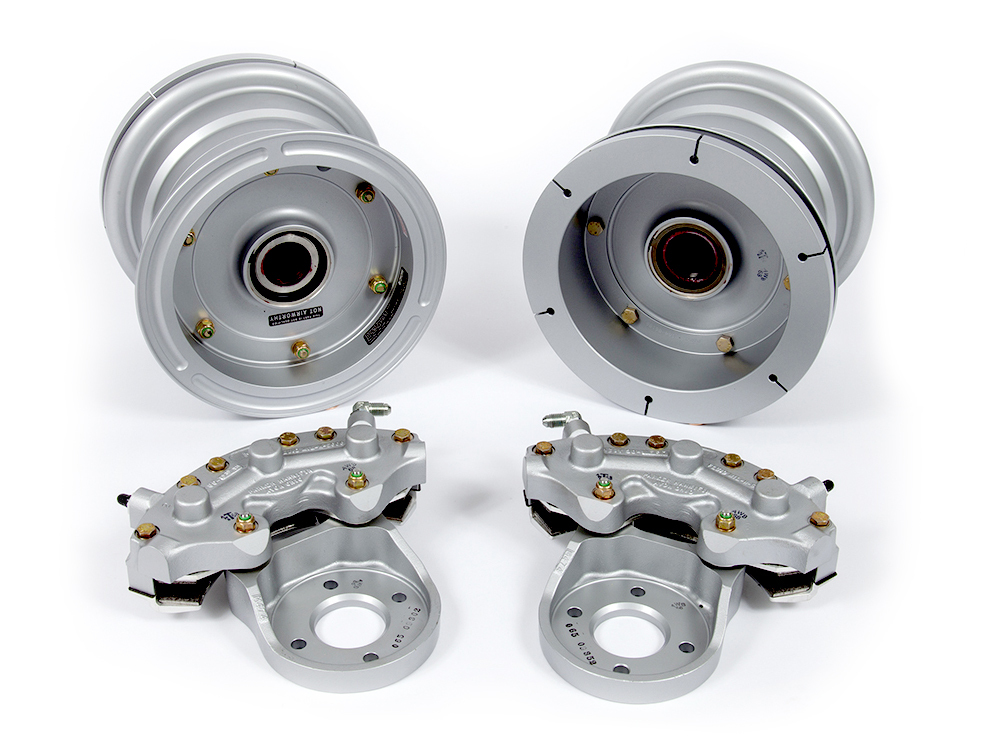The image depicts an assembly of intricate silver metal machinery parts against a white background. In the background, there are two cylindrical, silver-toned objects, each featuring a central circular section with various bolts or screws encircling the perimeter. The left object has a distinct black and white central area, while the right one displays a red and brown center. Each of these cylindrical objects appears to have extended sections at both ends, suggesting a layered, barrel-like structure.

In the foreground, positioned in front of each cylindrical object, are two similar metal components that resemble brake calipers. These components, likely part of a Cleveland Brakes main wheel and brake kit, feature curved, C-shaped structures with copper or brass-colored screws and fasteners prominently visible. Each caliper-like component has a metal raised plate with embossed text, unreadable due to the image quality, and several additional screws securing the assembly. The base section of these components includes a round bowl or depression, flat at the bottom with a central hole, giving them a distinct depth and form. The precise arrangement and repetitive design elements, coupled with the detailed fastenings, suggest a robust and functional mechanical assembly designed for precision and stability.